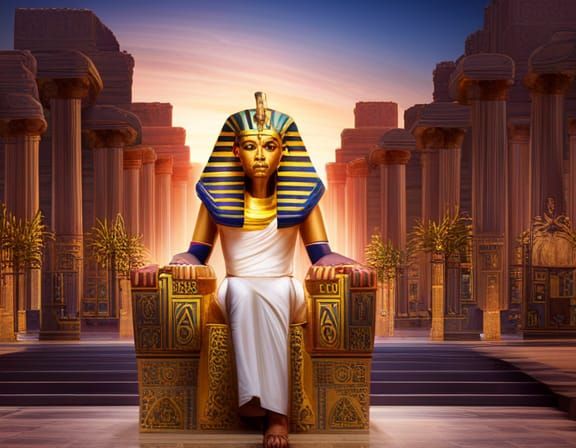The image depicts an Egyptian pharaoh, centrally located and seated on a bronze, golden throne intricately designed with a hard metallic appearance. The pharaoh, with a darker skin tone, is adorned in a traditional white robe along with brown sandals and a gold neck collar. He wears an iconic Egyptian headdress marked by blue and gold stripes, with some stripes running horizontally and others vertically, accentuating his golden mask-like face.

The background reveals a majestic architectural setting, featuring marble columns on both sides of the pharaoh that extend high upwards. These columns are sand-colored with detailed gold carvings at their bases. Small plants are placed near the base of these columns, adding to the grandeur. Behind the pharaoh, a pathway lined with these columns leads towards glowing light, suggesting the sun either rising or setting, bathing the sky in a warm hue contrasted by patches of a blue sky. Steps ascending from the back of the throne further emphasize the regal and ancient Egyptian atmosphere of the scene.